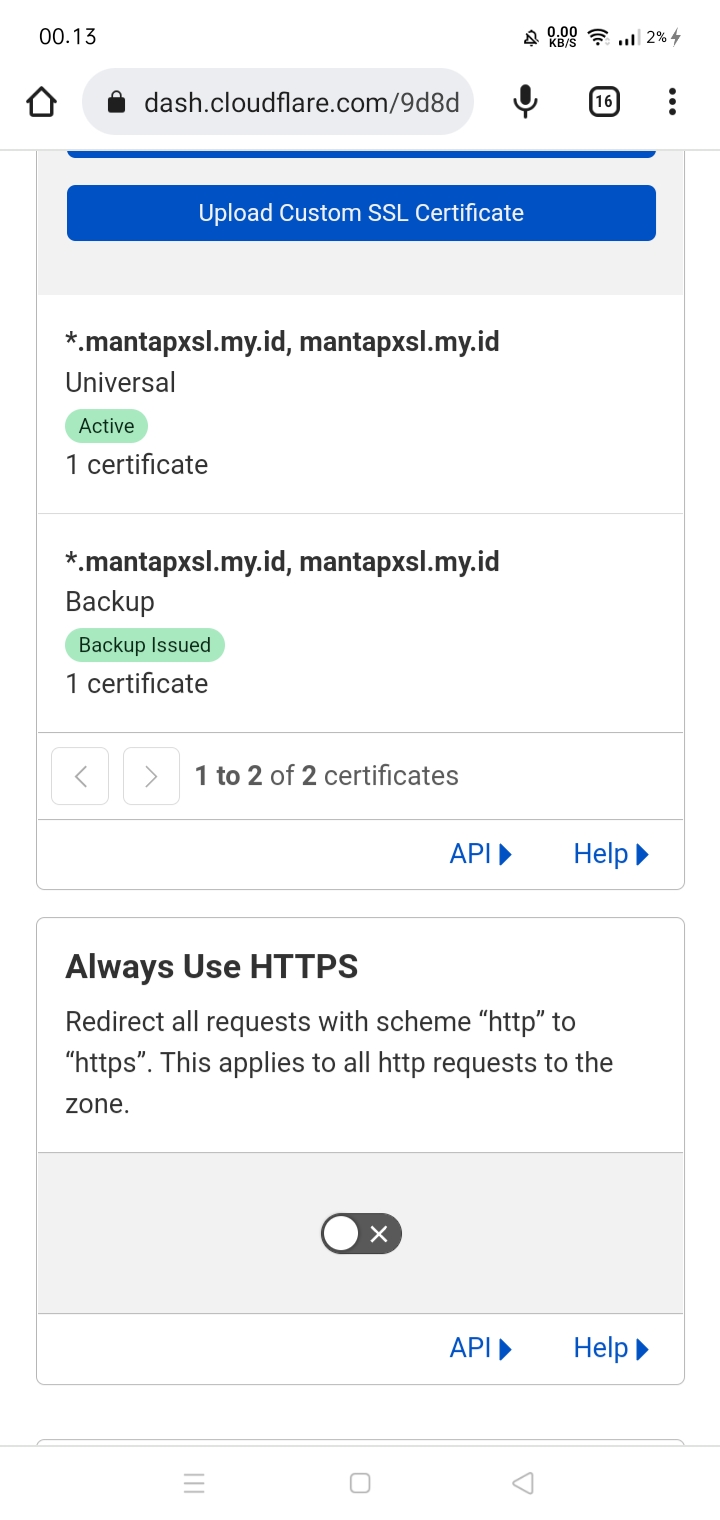The image is a detailed screenshot taken from a cell phone, displaying a web page from the URL "dash.cloudflare.com/9d8d." At the top of the screen, the timestamp reads "00:13," and there are several status icons, including a bell, settings, a KB/s indicator, and Wi-Fi signals with ascending bars. Notably, the battery area shows "2%" alongside a lightning bolt symbol, indicating the phone is charging.

The web page features a blue rectangular button with curved edges, labeled "Upload Custom SSL Certificate." Below this, there is a section containing a link labeled "Universal" and the status "Active" inside a green circle. Additionally, there's another "Active" status within a green circle for "Backup Issue." At the bottom of the screen, there's an option labeled "Always Use HTTPS," which is currently turned off.